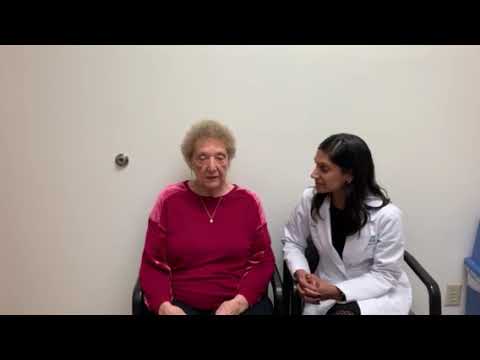In the photograph, two women are seated side by side in a room. The woman on the left, who appears to be elderly and over the age of 60, is wearing a red sweater with pink shoulders and black pants. She has short, blondish-brown hair with hints of gray, and she has a tiny gold necklace around her neck. Her expression is sad and serious as she looks down with her hands resting in her lap. The woman on the right appears to be a doctor, dressed in a white medical coat over a black blouse. She has olive skin and long black hair that cascades over her shoulders. Her hands are clasped together in front of her, and she is slightly turned towards the elderly woman, looking at her with a concerned expression. Both women are seated in black chairs. Behind them, the wall is white with a door stopper visible on the left side. In the bottom right corner of the image, there is an electrical outlet and what looks like the edge of a blue trash can. The overall mood of the scene is mellow, with both women displaying subdued emotions.